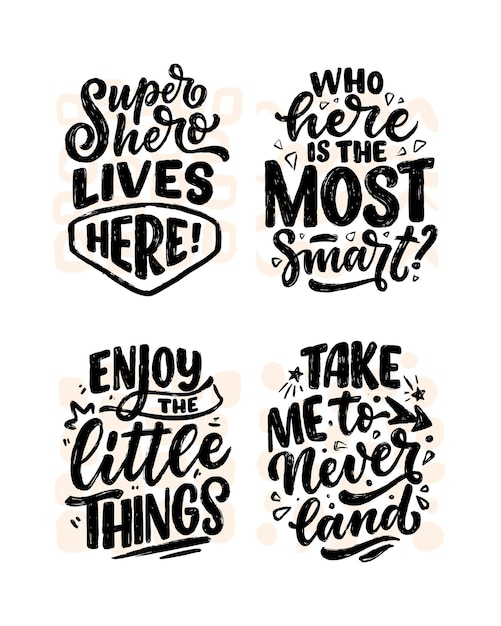The image features four distinct motivational sticker designs, each enclosed within an oval shape and accentuated by a shadowy peach background. The top-left design reads "Superhero lives here," with "Superhero" in cursive and accented by confetti-like drawings. To its right, the second design poses the question, "Who here is the most smart?" with "here" and "smart" elegantly written in cursive, surrounded by confetti and ornamental details. Below that, on the left, is a design that says, "Enjoy the little things," where "little" is rendered in cursive script. Finally, the bottom-right design reads, "Take me to Neverland," with "to Neverland" in cursive, accompanied by illustrations of stars and an arrow. Overall, the text is presented in a mix of cursive and bold fonts, adorned with decorative elements like shooting stars and diamonds to enhance visual appeal.